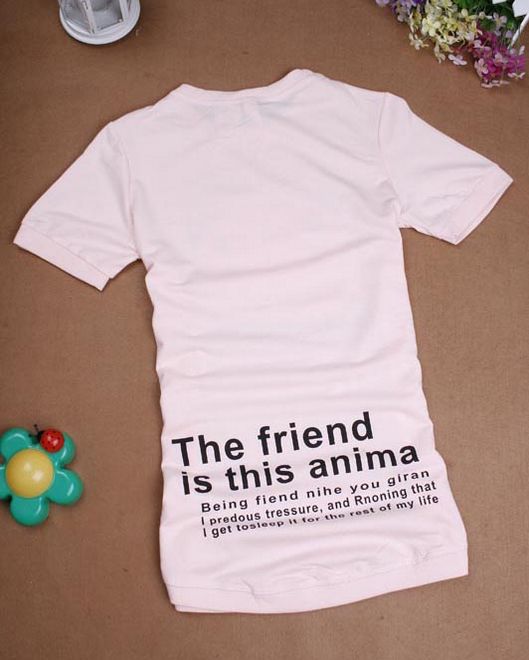The image displays a white, men's crew neck t-shirt lying flat on what appears to be a brown tile or carpeted floor. The t-shirt has some ripples around the body area, and features a bolded black text across the bottom that reads, "The friend is the enema". Beneath this, in smaller, left-aligned black text, is a nonsensical string of words: "being fiend, near you, Geron, I prejudice Tresha, and knowning that I get to sleep it for the rest of my life."

To the lower left-hand side of the t-shirt, there is a toy flower with a big yellow center and turquoise petals, decorated with a ladybug on one of the petals. In the upper right-hand corner of the image, there are some purple and yellow flowers, which could be either artificial or real. Additionally, a small white object can be seen in the top left-hand corner.